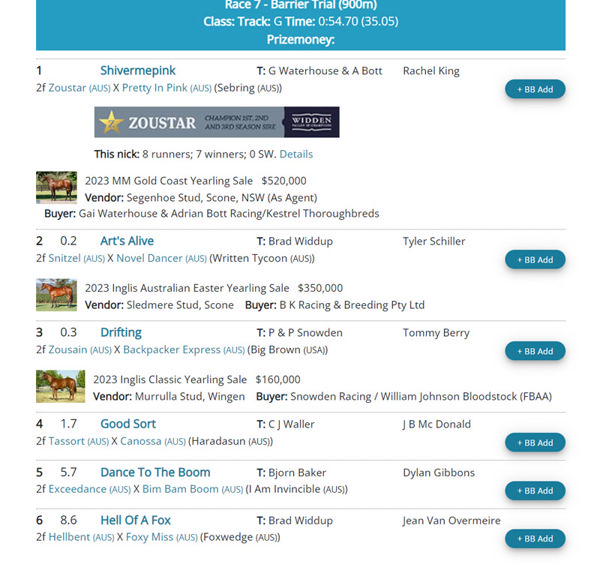The image displays a segment of a website, prominently featuring a blue banner at the top with centered text. The banner reads "Race 7 - Barrier Trial (900m)," followed by details such as "Class:", "Track: G", "Time: 054.70 (35.05)," and "Prize Money:". Below this header, on the left side, there's an entry labeled "1," next to which the text "Shiver Me Pink" is displayed. To the right of this, it reads "T: G Warehouse" and "Bot:", followed by "Rachel King." 

Further details mention the horse "Pretty In Pink (AUS)" just beneath the main entry. On the far right of the screen, there's a button labeled "BB Ad," accompanied by a banner. Below this, an image of a horse appears, with text indicating "2023 MM Gold Post Year-End Sale, 520,000," along with additional information pertaining to the sale.

Following the initial entry, there are similar sections labeled "2," "3," "4," "5," and "6." These entries, however, do not include images or media of horses. The design and format remain consistent across these sections, maintaining the structure of information seen in the first entry.